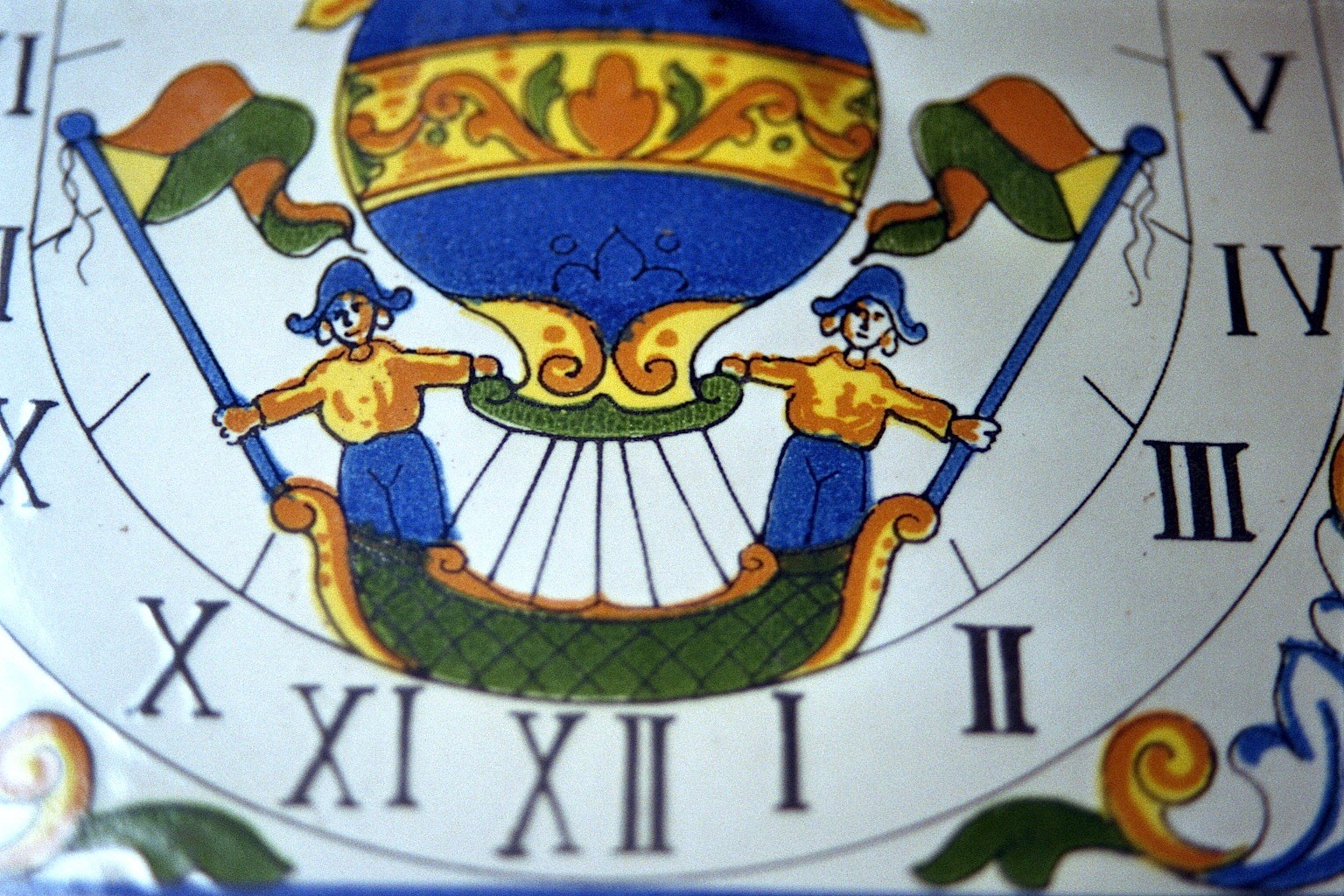This close-up image captures the bottom half of a clock face with Roman numerals displayed in an unusual order, suggesting the image may be flipped horizontally. On a white background, the Roman numerals run along a U-shaped border with XII at the bottom, followed by XI, X, and so on, to I on the right. Central to the image is a detailed depiction of a hot air balloon lifting a boat. The green boat features gold trim and spiral edges, and its basket holds two women dressed in blue pants, gold shirts, and blue sailor hats. They each hold blue poles adorned with pennants featuring yellow triangles near the poles and stripes of orange and green. The women's flags face each other. The scene is flanked on either side by partial leafy motifs, echoing the ornate spirals on the boat.